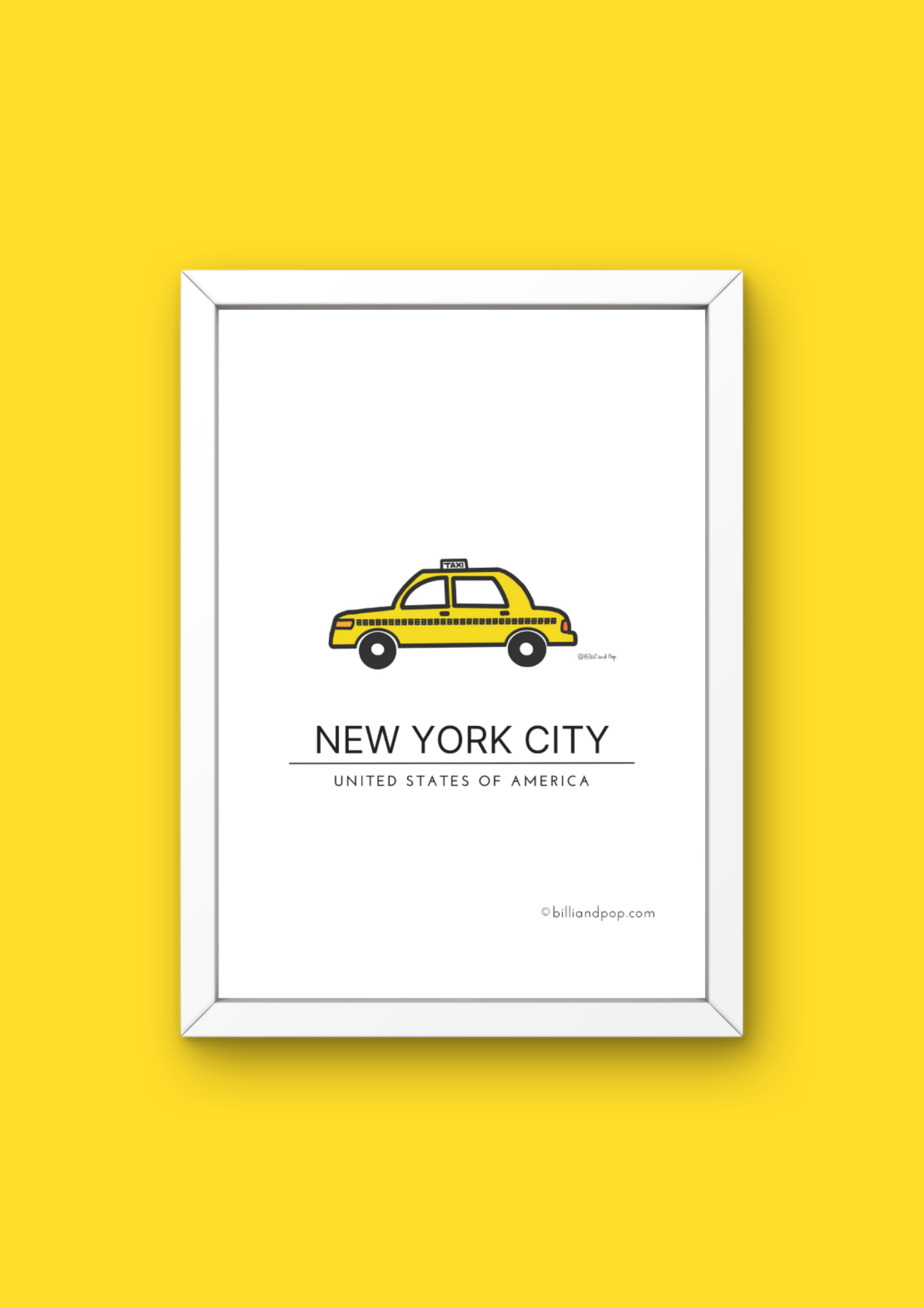The image presents a striking illustration set against a vibrant yellow background. Centered on this yellow backdrop is a white-framed poster, which features a simplistic cartoon drawing of a New York City yellow cab adorned with a black checkered stripe running from the headlight to the taillight. This empty taxi, depicted in a clip-art style, has a small rectangular "TAXI" sign perched on its roof. The cab is rendered with a clean, minimalist design, including circular black wheels.

Beneath the cab illustration, the words "New York City" appear in bold black letters, followed by a thin horizontal line. Directly below this line, the text "United States of America" is inscribed in a smaller yet matching black font. The backdrop of the poster maintains a white simplicity, framed by a whitish, almost silver border approximately half an inch thick. Lower down and to the right of the taxi, near the brake lights, there is a partial and barely legible website credit that reads "billiaandpop.com." This meticulous framing makes it appear as though the entire piece is hanging on the yellow wall itself, creating a visually compelling and cohesive artwork.